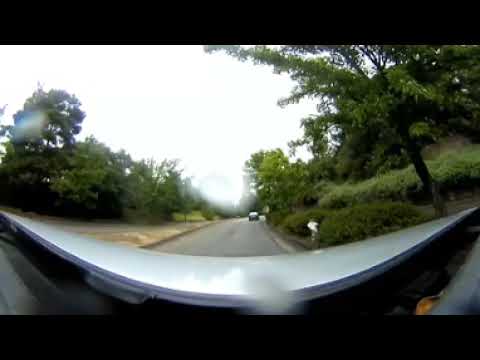The image captures a perspective from inside a vehicle looking out onto a road. The photo is taken from a slightly elevated viewpoint, possibly from within a car or a motorcycle, suggested by the visible dashboard or fairing. In front, there's a gray car, positioned centrally on the road, which stretches ahead with other small, indistinct vehicles driving away. The hood of the vehicle taking the picture is gray, while the dashboard is black. The surroundings feature grassy areas and numerous trees, with hills gently sloping upwards on both sides of the road. On the right side, there's a road sign or speed limit sign, although the text is unreadable. The landscape appears lush with different shades of green and occasional spots of other colors like yellow and red. The day is extremely cloudy, the sky covered in a uniform layer of clouds that render it primarily white, devoid of blue patches or sunlight. The scene seems to be situated on a highway, with various objects such as road signs and lights, and the entire setting evokes a sense of travel through a verdant, hilly countryside on an overcast day.